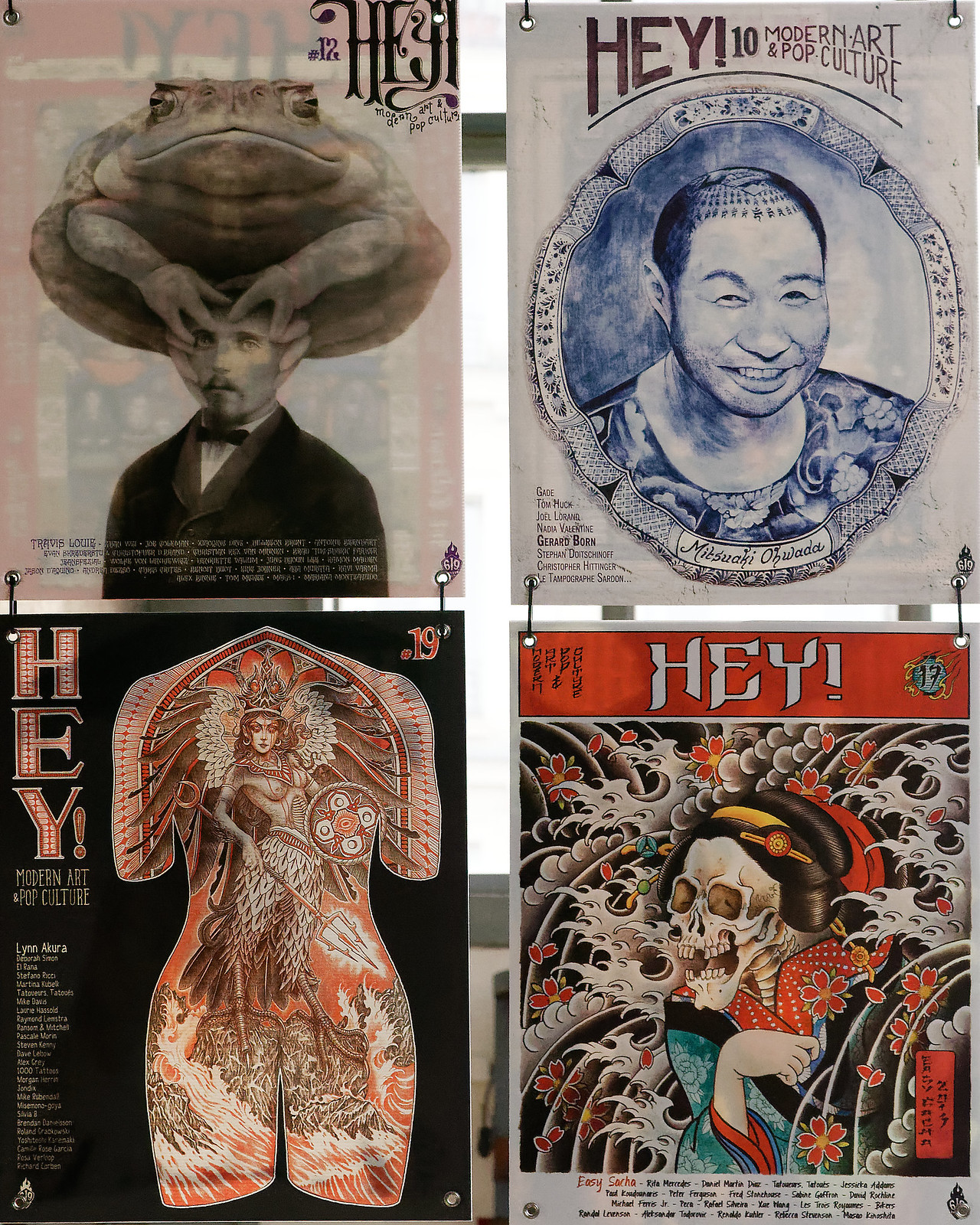The image depicts four artistic posters, arranged in a two-by-two grid, each adorned with distinctive and intricate designs, all under the common title "Hey" and varying numbers. 

- **Top Left Poster:** This grayscale poster features a surreal scene where a large, obese frog is perched atop a man's head, its limbs draped over him. The man, dressed in a tuxedo and bow tie, stares slightly leftward with a solemn expression. The word "Hey" and the number 12 are prominently displayed in the top right corner, with additional text across the man's chest.

- **Top Right Poster:** This is a colored portrait of a man with a bald head and elaborate tattoos extending from his forehead to his neck. His facial expression is calm, and he is surrounded by ornate flourishes. The title "Hey" along with "Modern Art and Pop Culture" is prominently displayed, along with the number 10.

- **Bottom Left Poster:** An intricate outline of a headless and limbless torso appears against a minimalistic background. Within the outline is a detailed illustration of a human-animal hybrid, with bird-like legs and expansive black wings. This figure holds a trident and stands upon a rock amidst water. The word "Hey" runs vertically down the left edge, accompanied by the number 19.

- **Bottom Right Poster:** A striking image of a geisha-like skeleton is depicted, with a fully detailed skull and a flesh-covered arm. The figure wears traditional attire, complete with an elaborate hairstyle pinned up. Surrounding the figure are artistic representations of waves and floral designs. The word "Hey" appears in large white letters with an exclamation point in a red border at the top.

The posters are artistically pinned together, two on the left and two on the right, with a narrow white space in between, potentially outlining the top and bottom of a window.